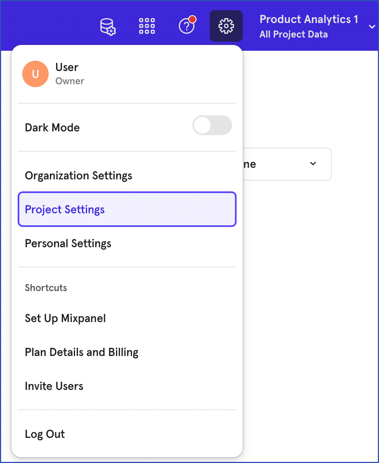The image displays a detailed interface of a web application with a distinct header and side menu. The top header features a background in a deep purple color with the text in white. In the top-right corner, it reads "Product Analytics 1, All Product Data." Adjacent to it on the left, there's a highlighted settings icon depicted as a white gear over a dark background. Proceeding leftward, there is a white help button marked by a question mark, which has a small orange dot above it to denote notifications. Next, there is an icon comprising nine white squares, followed by another settings icon with a cylindrical shape.

The side menu, opened on the left part of the image, begins with a section labeled "User, Owner," accompanied by an orange icon featuring a white "U" in the center. The icons in this section are well-defined. Below this section, there's an option labeled "Dark Mode," which is currently active as evidenced by the dark header and the predominantly white background of the image. 

The side menu continues with "Organization Settings" followed by "Project Settings," which is highlighted with a purple outline, indicating it is the selected option. Subsections under "Project Settings" include "Personal Settings," and "Shortcuts." Following these options, the menu lists "Setup Mix Panel," "Plan Details and Billing," "Invite Users," and at the bottom of the menu, there is a "Logout" option. The white background of the main content area contrasts with the dark header, adding clarity and focus to the interface elements.